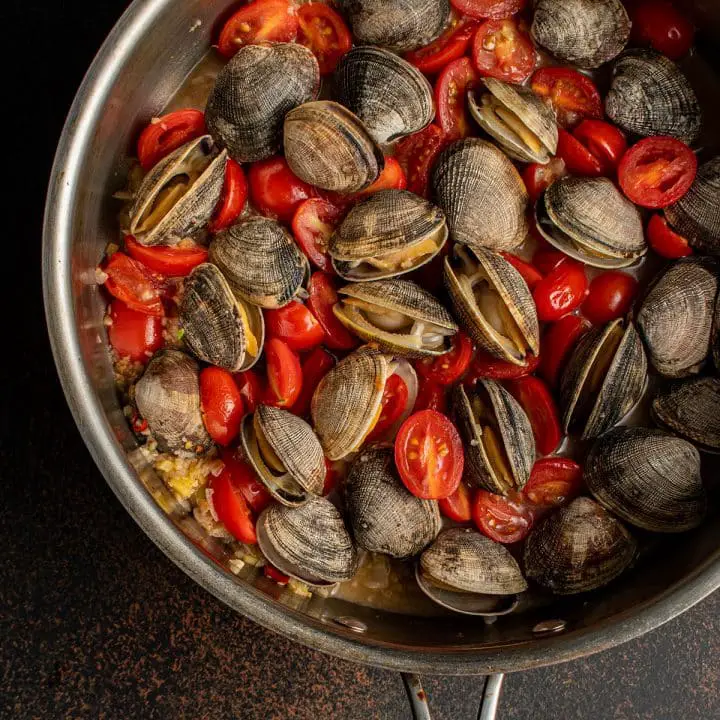In this overhead image, we see a large, slightly off-centered, silver metal pot or bowl taking up the majority of the frame. The pot is situated on a speckled countertop with black and rust hues, resembling a textured sponge-paint design. The backdrop is just the countertop, as no other elements are visible. 

Inside the pot, which is slightly cut off in the upper right corner, there are numerous clams in shades of black, white, and gray, some with striped patterns. These clams appear to be partially open, suggesting they might soon be cooked. Among the clams are small red tomatoes, sliced open, all immersed in a brownish liquid. The varied colors in the image include black, brown, gray, silver, red, and yellow tones, indicative of a kitchen or restaurant ambiance where a seafood dish like clam soup, gumbo, or jambalaya is being prepared.